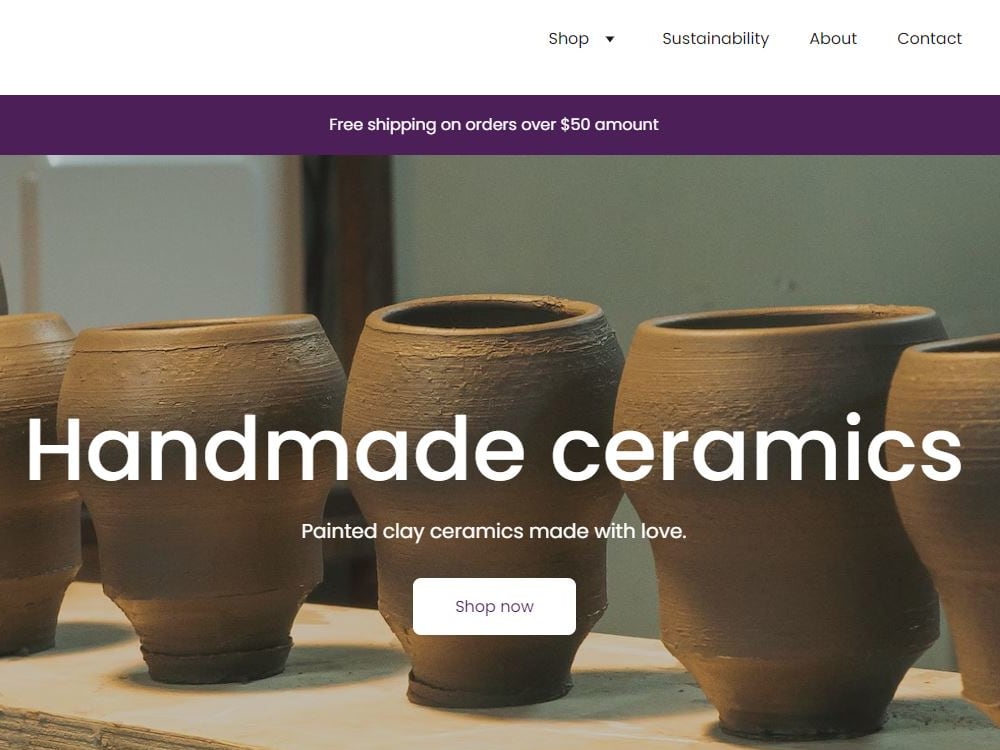The image is an advertisement for handmade ceramics, featuring a prominent banner at the top with a purple background and white text that reads "Free shipping on orders over $50." Below the banner, a row of brown ceramic pots is displayed on a white surface. The pots vary slightly in size and are arranged so that three are fully visible, while the other two are partially shown at the image's edges. Superimposed in white lettering across the middle of the image is the text "Handmade Ceramics," followed by "Painted clay ceramics made with love" in smaller font underneath. At the bottom of the image, a white rectangular button labeled "Shop Now" invites the viewer to browse and purchase the ceramics. Despite the caption mentioning "painted," the ceramics in the picture remain in their natural brown clay state.